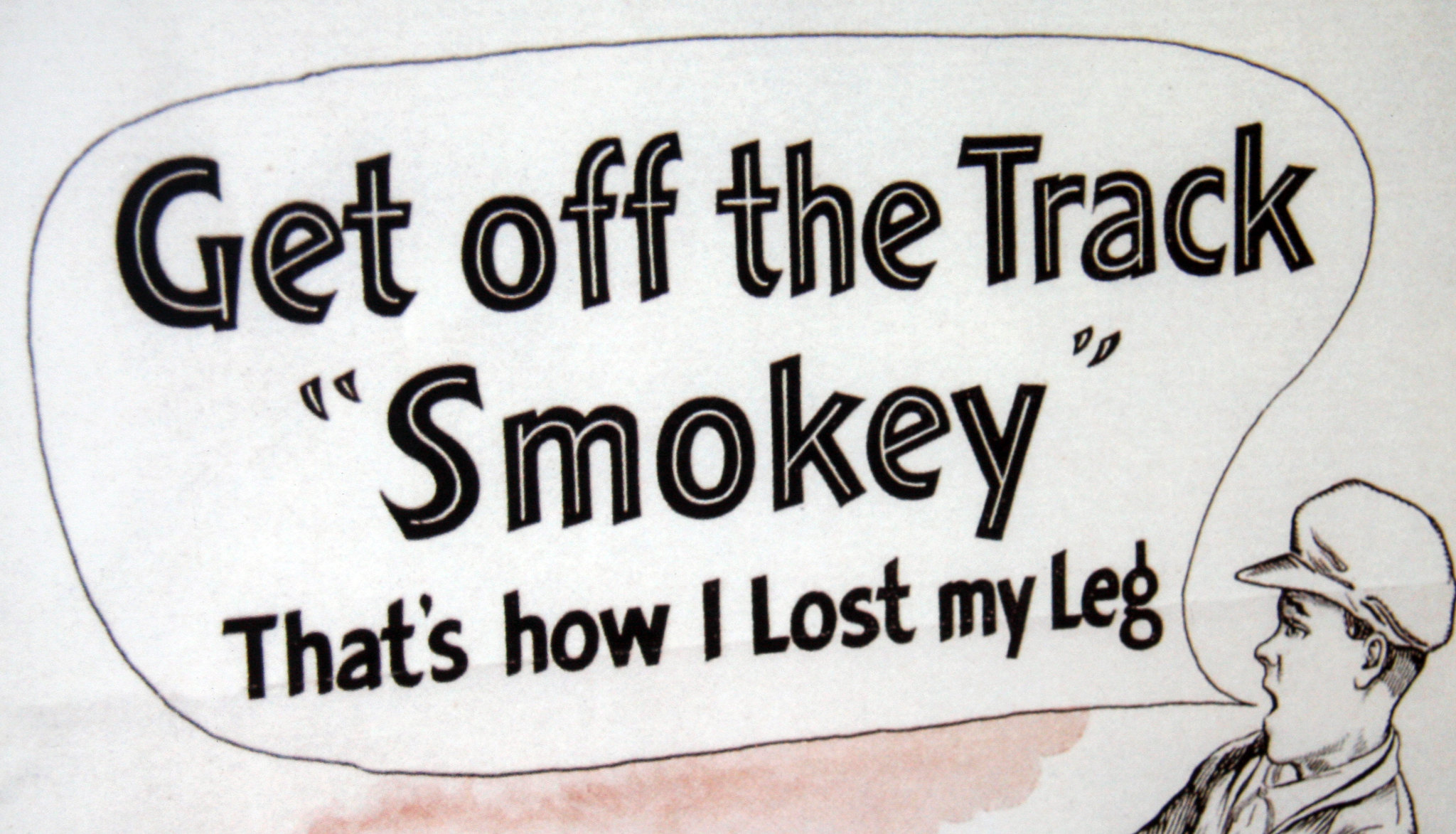This is a detailed photo of a pencil drawing, predominantly rendered in black. The drawing features a human character situated at the bottom right corner, who appears to be the focal point of this piece. This character, dressed in a collared shirt and wearing a cap that resembles a train conductor's hat, is speaking through a speech bubble. The text within the bubble is also in black and reads, "Get off the track, Smokey. That's how I lost my leg." The word "Smokey" is emphasized with quotation marks. The background is light gray, with noticeable blotches of pink color towards the bottom, which appear intentional as they neatly end at the edge of the speech bubble. This detail suggests that the pink shading is part of the original illustration and not a stain. Overall, the illustration evokes the style of an old advertisement or public service announcement, possibly found in a magazine, using a comic-strip-like format to convey its message.